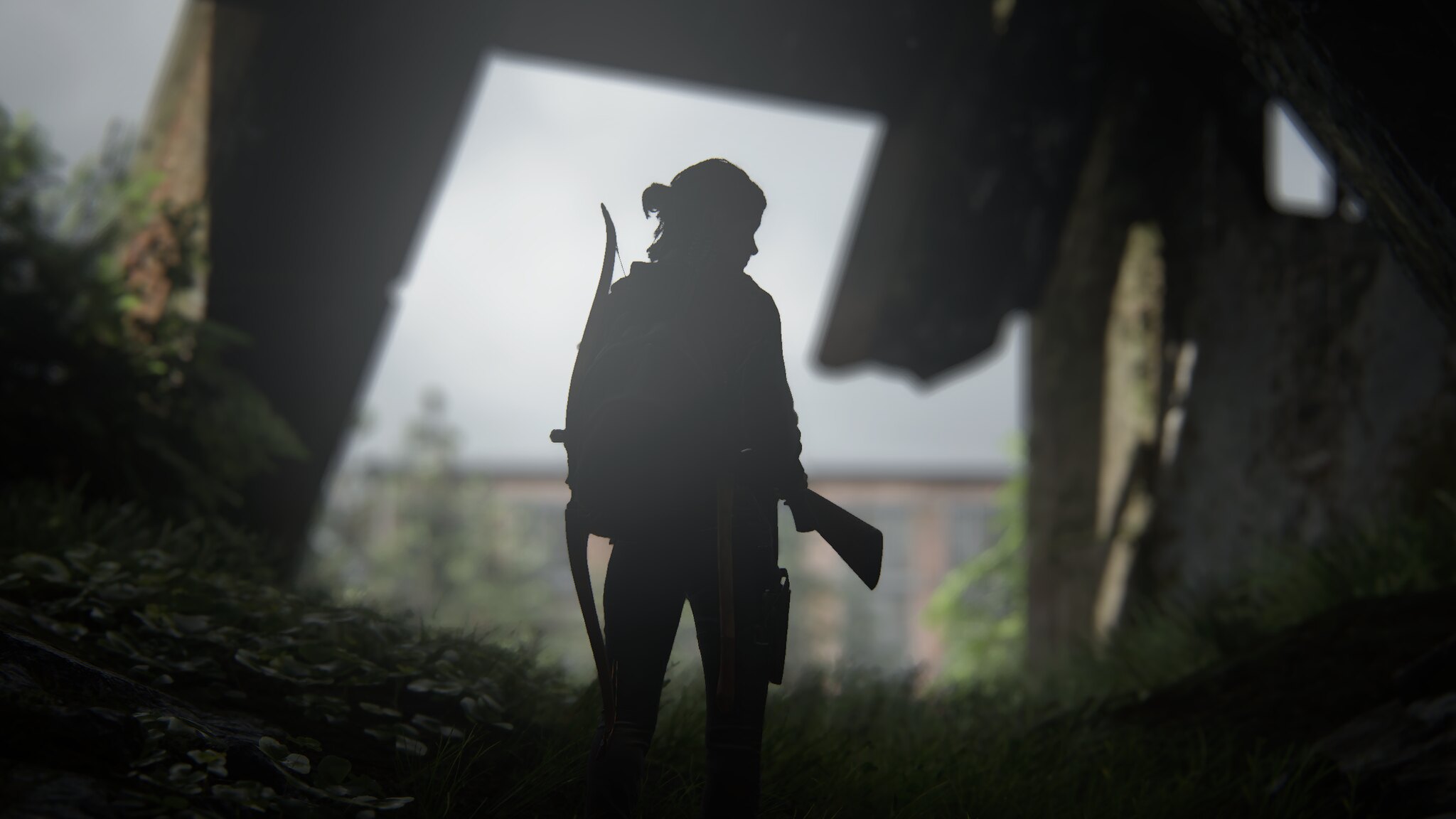The photograph is a color image with significant portions enveloped in shadow, lending it a dark, almost mysterious feel. It is a rectangular image oriented in landscape format, wider than it is tall. The perspective appears to be taken from behind some sort of wooden structure, possibly a building, framing a view of the outside world through an opening.

In the center of the composition, there is the silhouette of a person, their features obscured by the shadows. Despite the lack of detail, you can discern that they are standing upright, visible from the knees up, and possibly have a ponytail, as suggested by the shape at the back of their head. The figure is looking to the left.

Behind this figure, the sky is bright blue, contrasting sharply with the darkened foreground. To the right, part of a building is visible, albeit out of focus. The person appears to be equipped with various items: a bow and arrow slung over one shoulder and a gun on the other side, though the specifics are lost to the shadow.

The overall composition creates a stark juxtaposition between the dimly lit interior and the brightly lit exterior, enhancing the enigmatic nature of the silhouetted figure positioned centrally in the frame.